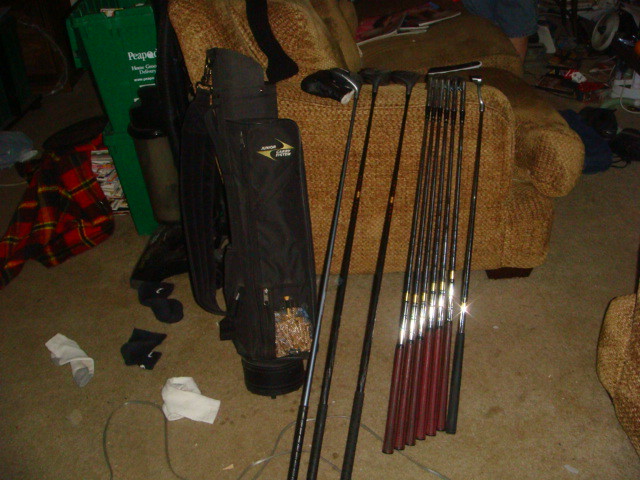In this dimly lit, indoor photograph, we observe an untidy room dominated by a collection of golf equipment. A set of well-used golf clubs, both with black and red grips, stand vertically with their heads resting against the side arm of a profile-visible armchair. This chair is upholstered in a light brown or pale rusty fabric. Adjacent to the golf clubs are black golf club bags featuring indistinguishable logos and symbols. The floor, covered in a dirty brown carpet, is scattered with various items including a pair of white socks, tissues, and wires. To the left, a plaid red and black afghan is crumpled up in a heap. The overall setting suggests a cluttered and scruffy living space, enhanced by the presence of scattered magazines on the arm of the chair and additional unidentified items on the floor. The poorly lit and slightly out-of-focus image accentuates the disordered ambiance.